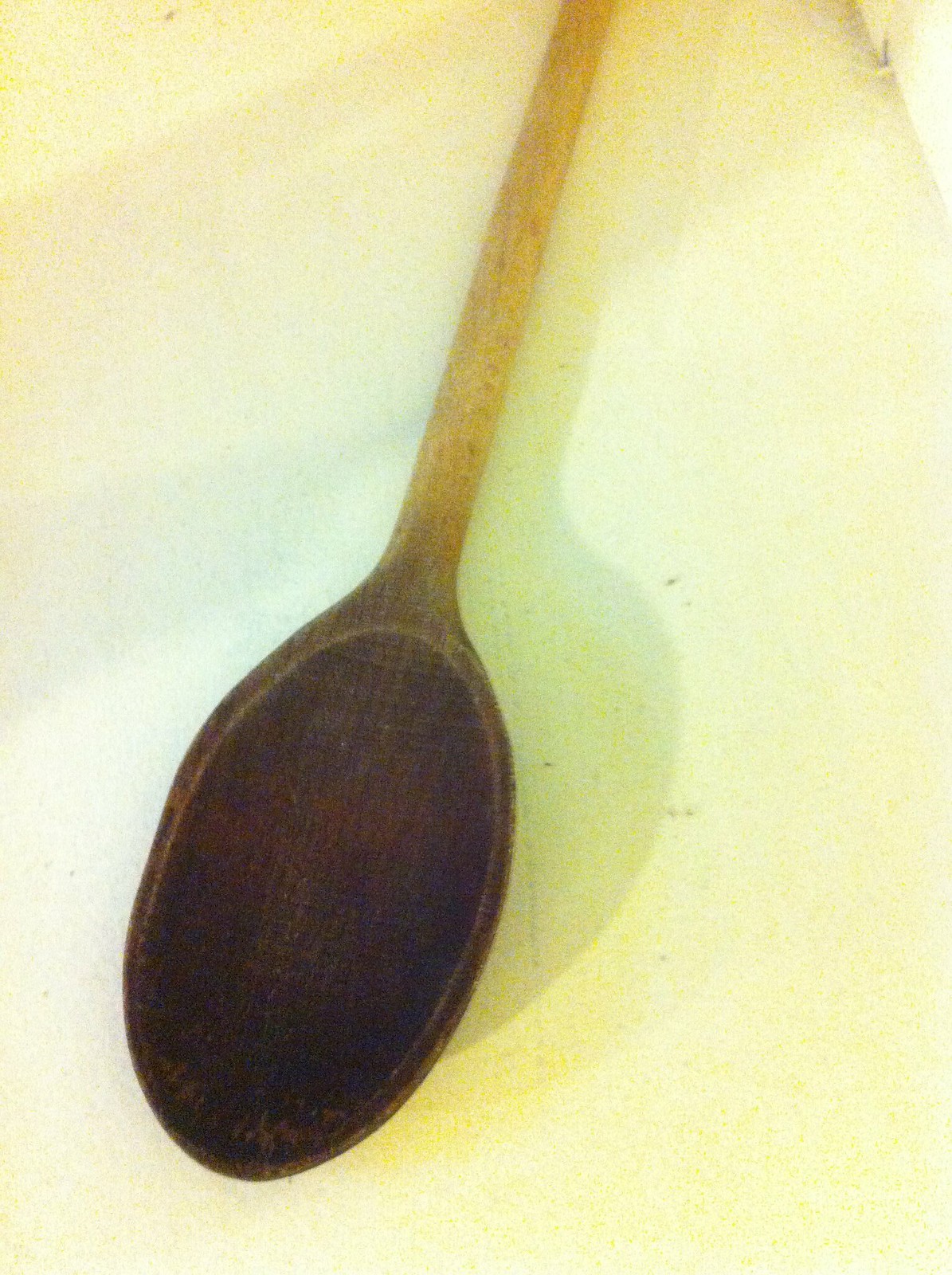The image captures a well-used, older wooden spoon with a dark brown head and a lighter brown handle extending about four to five inches into the frame. The spoon is positioned diagonally on a light cream-colored surface that has hints of yellow and blue in the shadows, giving depth to the image. The spoon casts a shadow onto the surface, reflecting the underlying hues. Despite appearing somewhat blurry, possibly due to being taken with a mobile phone camera, the details of its wear are evident. The spoon's darker head suggests frequent use in stirring darker liquids, such as teas. The overall composition lacks any additional elements like people, buildings, or vehicles, focusing solely on the spoon against the nuanced background.